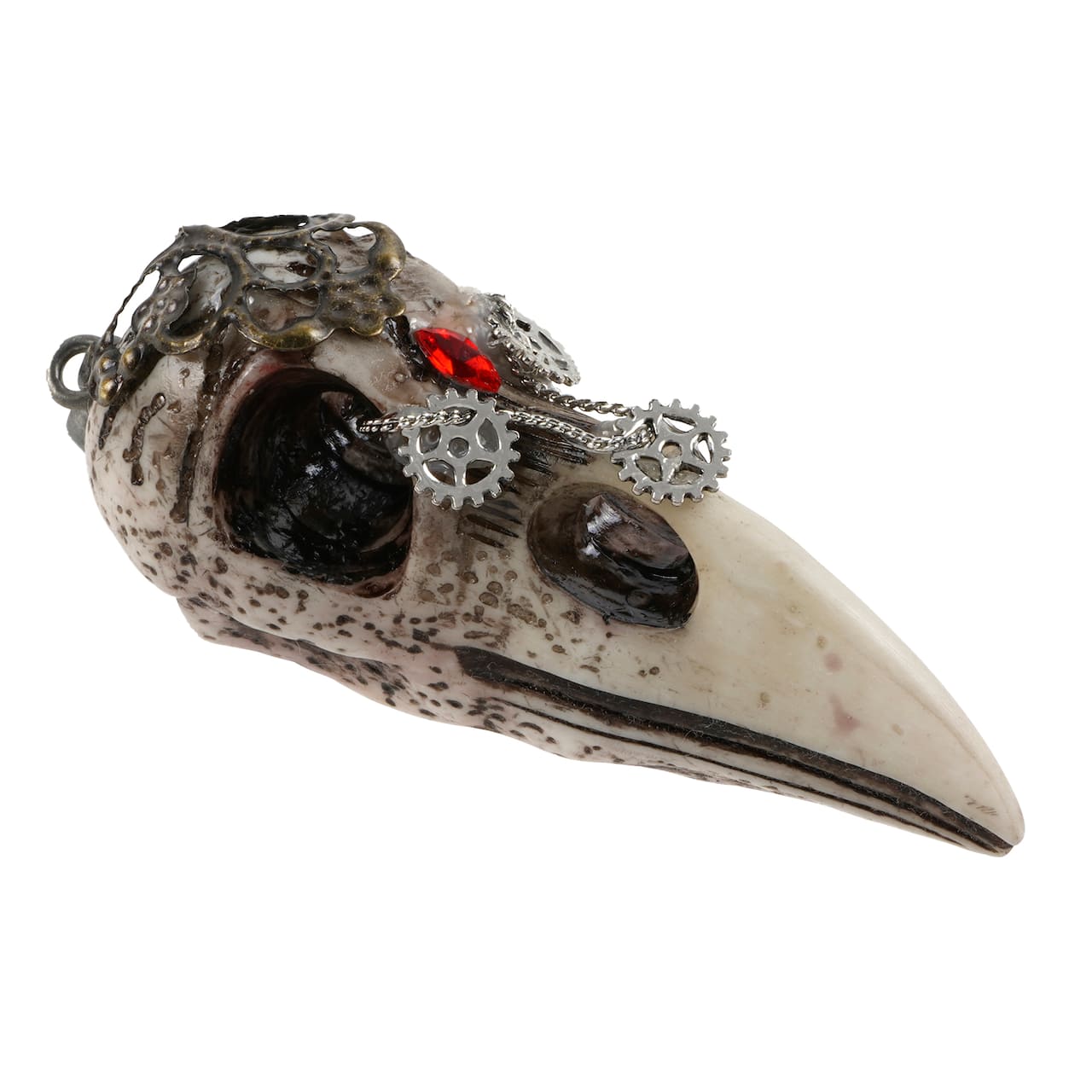The photograph depicts an ornately decorated bird skull with a distinctly eerie appearance, set against a stark white background. The skull itself is off-white in color, resembling ivory or bone, and features prominently large, hollow, and blackened eye sockets along with a long, curved beak. Grayish pits mar its surface, particularly towards the head and eye regions. The most striking elements of the decoration include several metal chains looped over the top of the skull and through the eye sockets. The chains are crafted from goldish and silver metals, contributing a steampunk vibe to the artwork. A prominent red stone, diamond or oval-shaped and resembling a ruby, adorns the center of the skull. Below this stone, three metallic gears are interconnected by a silver chain, with one gear positioned on each side of the skull and another extending down towards the beak. Additionally, there is a large brown oval area on the beak, adding to the skull’s unsettling aesthetic. The combination of these mechanical and jeweled elements gives the piece an intricate, almost necklace-like appearance, enhancing its eerie, yet intriguing, allure.